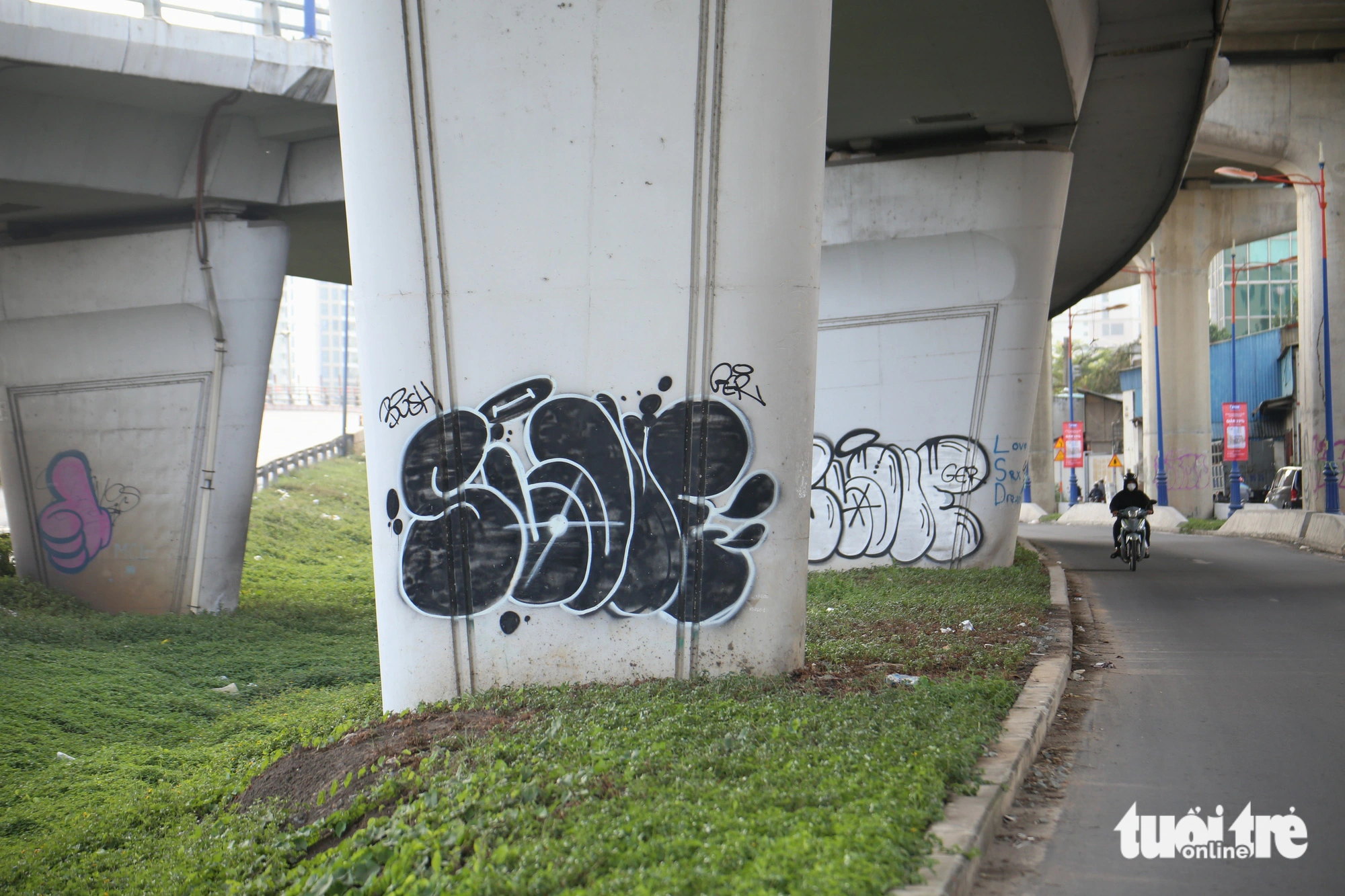The photograph is a clear, brightly taken image of a cityscape, captured from underneath a curved on-ramp or off-ramp bridge. The urban scene features the infrastructure of multiple bridges, displaying both older suspension elements and newer, wider concrete columns supporting different roadways. In the foreground, there are large, squat pillars adorned with graffiti, including a prominent pink thumbs-up hand with three fingers. Two of the columns bear additional graffiti with partially decipherable text, one in black and another in white, possibly reading "Slive" followed by an inscrutable "T-O-U-I-T-R-E online." A green grassy area lies beneath the concrete structures. To the right of the image, a person rides a motorcycle towards the viewer along a road or alleyway, set against the backdrop of a heavily built-up, populated urban environment.